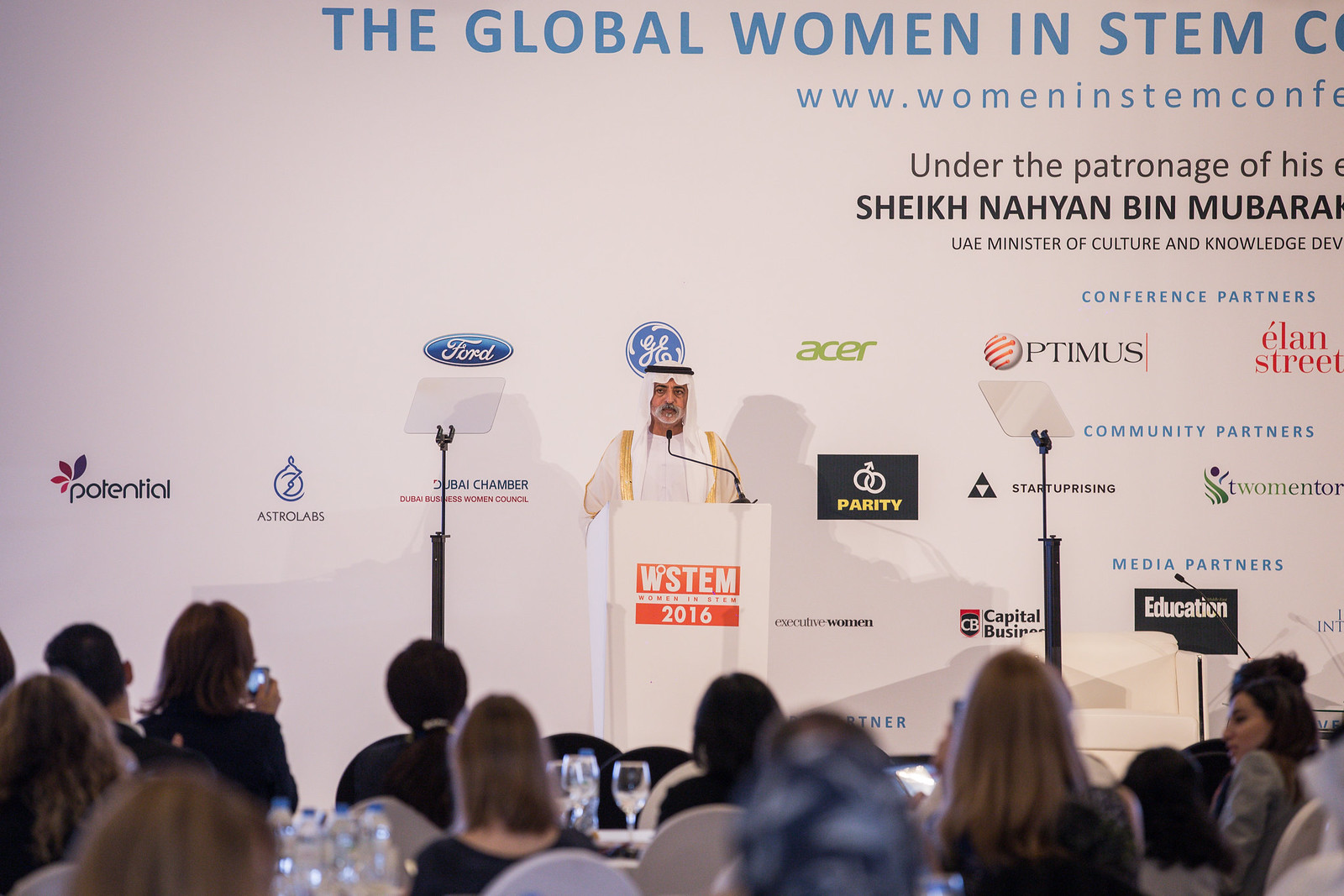The image captures a scene from the Global Women in STEM Conference 2016, held under the patronage of Sheikh Nayan Bin Mubarak Al Nahyan, UAE Minister of Culture and Knowledge Development. At the center of the frame, a man of Arab descent, dressed in traditional white Arab attire with a gold border and a black-ringed headdress, stands at a white podium adorned with an orange rectangle that reads "WSTEM 2016." The backdrop features numerous logos of conference partners, including Ford, GE, Acer, Optimus, and others, set against a white wall. The event details, including the URL www.womeninstemconference, are displayed prominently. The audience, predominantly women, are seated at white-covered tables, attentively listening to the speaker. Bottles of water and various glasses are visible on the tables, and some attendees sport head coverings.